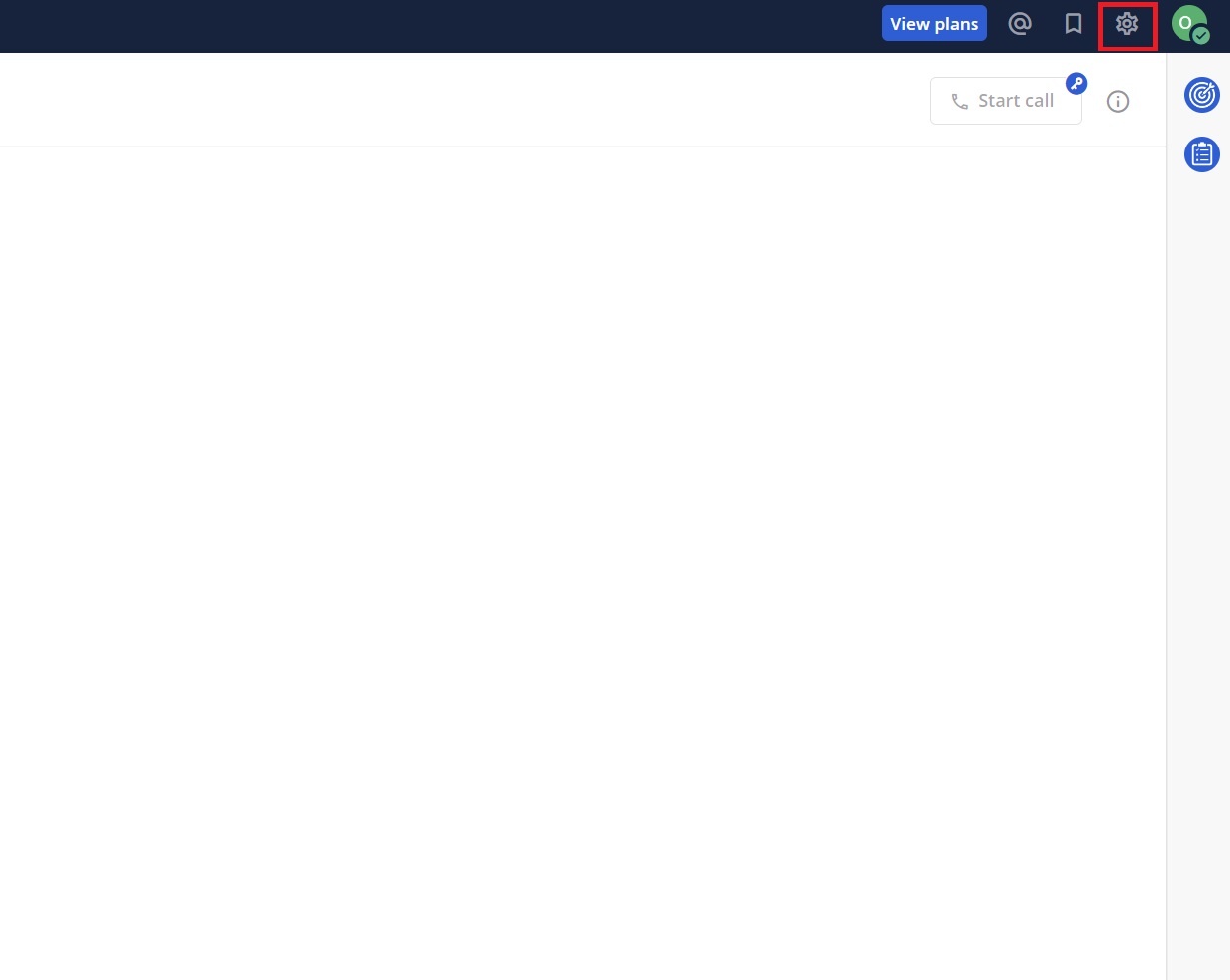A screenshot of a website interface with a predominantly blank central area. At the top, there is an elongated black header spanning the width of the screen, empty except for the right side. Here, within the header, is a blue rectangular button with white text reading "View Plans." Adjacent to this is a gray clickable area, followed by a gray ribbon-shaped icon, and then a gear icon encased in a red square suggesting it's an actionable item. 

On the extreme right end of the header, there is a white letter "O" inside a green circle, a smaller green circle with a checkmark beneath and beside it. Further down the page, a faint green-gray line extends across, terminating near some text that reads "Start Call" alongside a small gray phone icon. The upper corner features a blue circle, and down the right side of the screen, there are two other blue circles aligned beside a gray vertical line running down the screen's right edge.